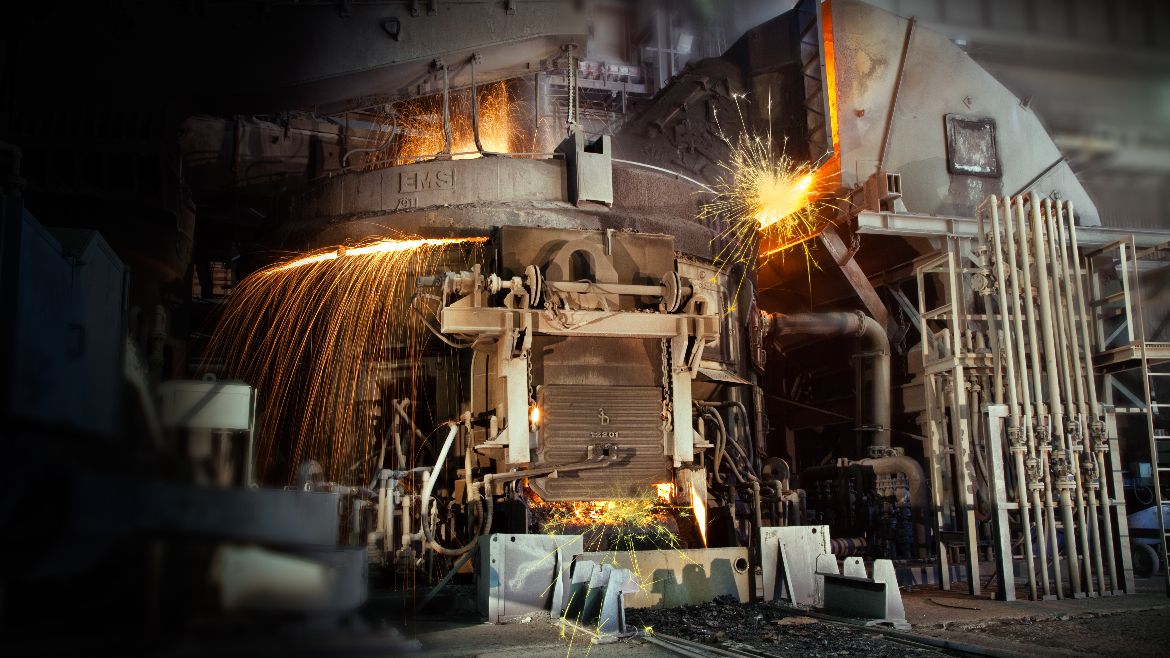The high-resolution photograph captures a scene of an industrial process within a factory setting, focusing on a large, complex machinery. Dominating the center is a cylindrical structure with a heavy lid pressing down, emitting bright sparks indicative of a high-temperature process, likely welding or molten metal work. This structure appears to be constructed from grayish metal with a cement-like base. Prominently displayed on the structure is a door labeled "12201" with sparks bursting from its edges. Above the door, the marking "E.M.S." is faintly visible along with some illegible numbers. The left side of the image is darker and features gray metallic components, while the right side showcases a network of vertical metal rods and pipes, extending upwards from the floor and arching into the machinery, suggesting an intricate system of supports and conduits. The photograph vividly captures the intensity and complexity of industrial fabrication work.